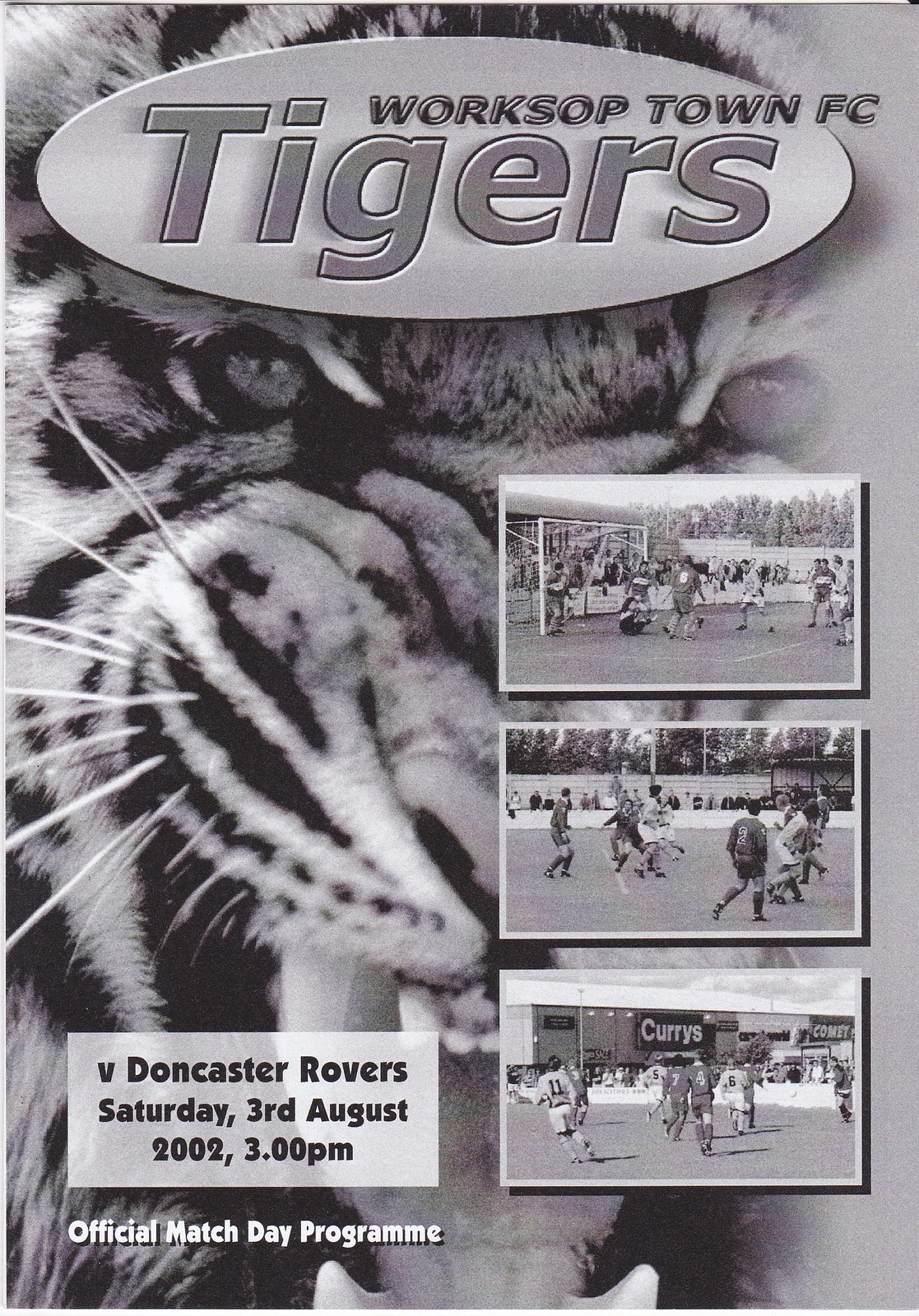This is a tall rectangular black and white flyer featuring a super zoomed-in image of a roaring tiger's face as the background. The tiger's eyes are positioned just above the middle of the image, and its open mouth, showcasing sharp teeth, is at the bottom. At the top of the flyer, a wide sideways oval contains the text "Workshop Town FC Tigers" in dark gray letters. On the right side, three wide black and white photographs of soccer players in action are stacked vertically, each with a white border and a black shadow on the bottom and right sides. The bottom left corner of the flyer includes a transparent gray rectangle with black font that reads, "V. Doncaster Rovers, Saturday, 3rd August 2002, 3:00 p.m." and below it, in white text, "Official Match Day Program."